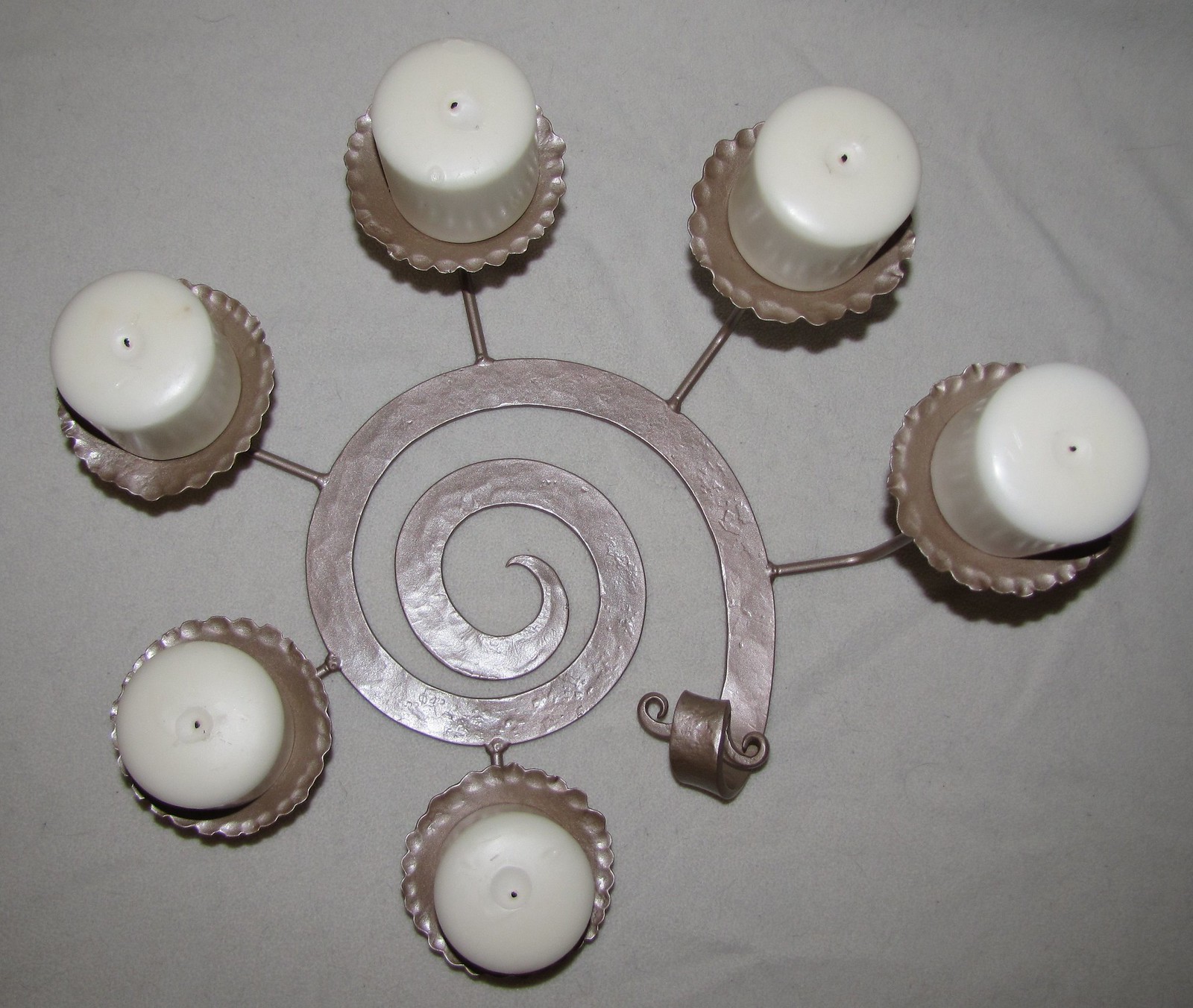This muted color photograph, likely taken in either pure or poor light, features a unique spiral candlestick holder with a winding, snail shell-like design crafted from a thin, bent brown metal. The base of the holder starts as a curved, ribbon-like metal strip that flattens out before swirling into a flat spiral. Attached to this central spiral are six (though one description mentions five) brackets that jut outwards, each forming a cup area with a rope or scalloped design around the edge. Each of these holders cradles a round, white cylinder candle, which notably appear unused and unlit as they lack blackened wicks. The background seems to be a white cloth with subtle ripples, adding a textural contrast to the scene. The spiral design of the holder causes the placement of the candles to be unevenly spaced, more spread out towards the top as the spiral expands.